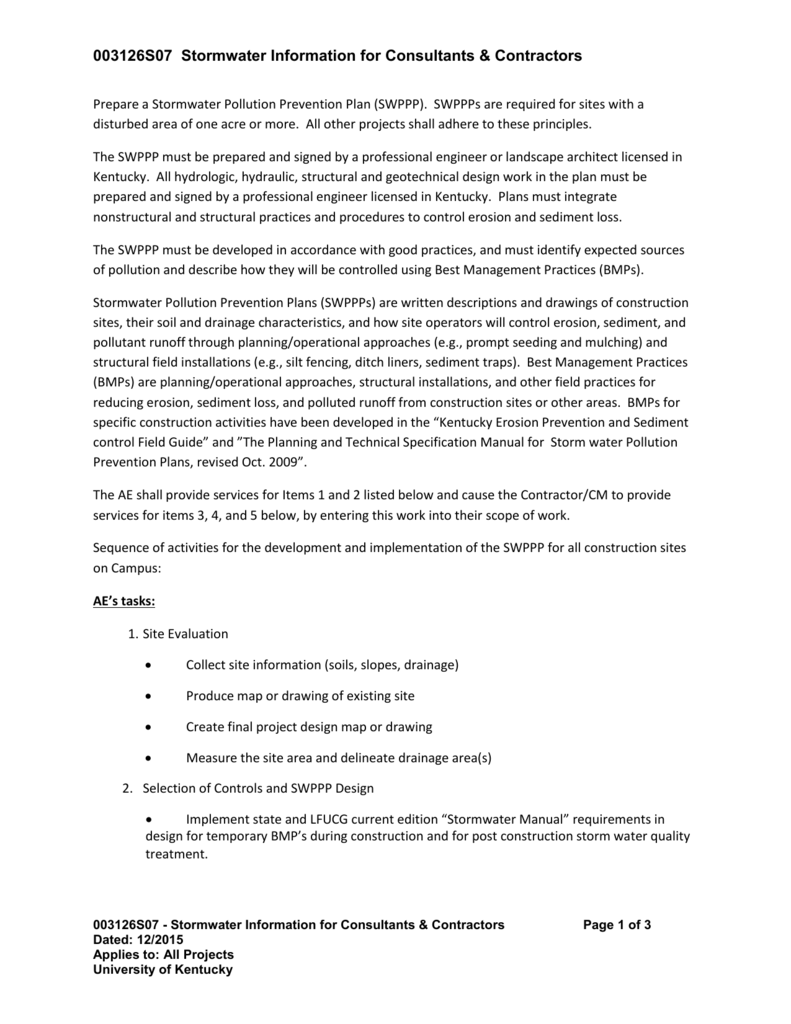**Website Detail: Stormwater Pollution Prevention Information for Consultants and Contractors**

Welcome to our website dedicated to providing essential stormwater pollution prevention information tailored for consultants and contractors. Below, you'll find a comprehensive guide to preparing a Stormwater Pollution Prevention Plan (SWPPP).

### Stormwater Pollution Prevention Plan (SWPPP) Requirements:

- **Scope:** SWPPPs are mandatory for sites with disturbed areas of one acre or more. All other projects must also adhere to the principles of effective stormwater management.
  
- **Preparation and Authorization:** The SWPPP must be prepared and signed by a professional engineer or landscape architect licensed in Kentucky. This also includes all hydraulic, hydrologic, structural, and geotechnical design work.

- **Content and Principles:** The SWPPP should integrate both non-structural and structural practices and procedures to control erosion and sediment loss. It must be developed in accordance with best practices and identify expected sources of pollution. The plan should detail how these sources will be controlled using established Best Management Practices (BMPs).

### Components of a Stormwater Pollution Prevention Plan:

- **Written Descriptions and Drawings:** The SWPPP must include written descriptions and detailed drawings of construction site characteristics, such as soil and drainage, and how site operators will control erosion, sediment, and pollution runoff through planning and operational approaches.

- **Best Management Practices (BMPs):** These include planning and operational approaches, structural installations, and other field practices designed to reduce erosion, sediment loss, and polluted runoff from construction sites. Specific BMPs have been developed and outlined in the Kentucky Erosion Prevention Sediment Control Field Guide.

### Roles and Responsibilities:

- **Architect/Engineer (AE) Tasks:**
  1. Site Evaluation:
     - Collect detailed site information.
     - Produce maps or drawings of the existing site conditions.
     - Create final project design maps or drawings.
     - Measure site areas and delineate drainage areas.
  
  2. Selection of Controls and SWPPP Design:
     - Implement the latest LFUCG (Lexington-Fayette Urban County Government) stormwater manual requirements.
     - Design for temporary BMPs during construction and ensure stormwater quality post-construction.
  
  The AE will also outsource specific tasks (items three, four, and five) to a contractor, integrating these responsibilities into the overall scope of work for the project.

### Documentation and Navigation:
- **Pagination:** This guide is part of a multi-page document. The current content represents page one out of three.

For further specifics on each of these components and to ensure compliance with local regulations, refer to the subsequent pages and sections of this document.